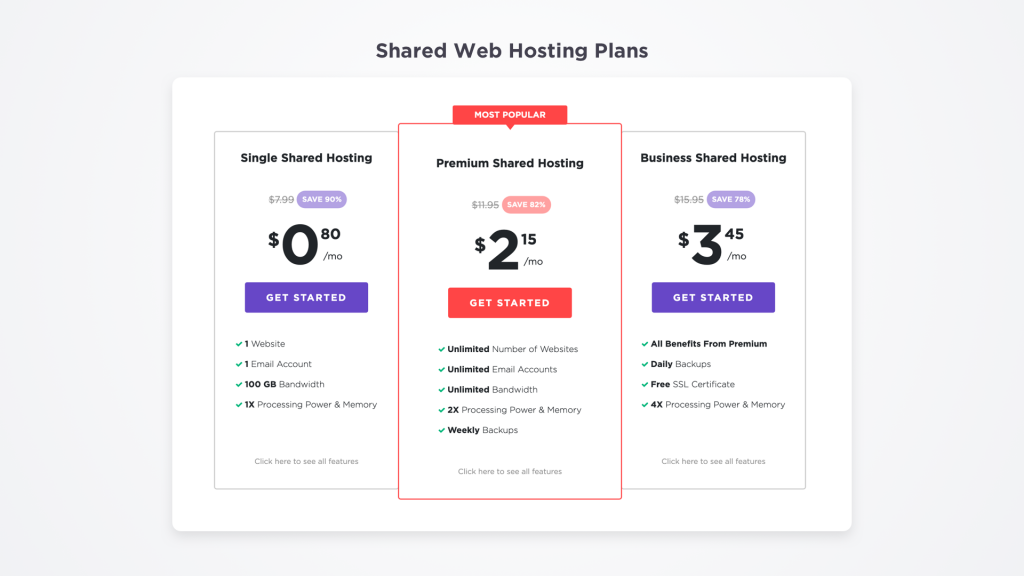This image is a screenshot displaying different shared web hosting plans within a larger light gray, vertically oriented rectangular box. Inside this box, the image itself has a white background and a title reading "Shared Web Hosting Plans."

There are three vertically oriented rectangular sections side by side. 

1. **Left Section: Single Shared Hosting**
   - **Price**: $79.99 is crossed out, and next to it in purple text, it states "Save 90%." 
   - **Current Price**: $0.80 per month with a purple "Get Started" button below.
   - **Features**:
     - One Website
     - One Email Account
     - 100GB Bandwidth
     - One Times Processing Power and Memory
   - Each feature is accompanied by a green check mark.
   - At the bottom, there's a clickable link, "Click Here to See All Features."

2. **Middle Section: Premium Shared Hosting**
   - This section is highlighted as the "Most Popular" with a red label at the top.
   - **Price**: $11.95 is crossed out, with a red text indicating "Save 82%."
   - **Current Price**: $2.15 per month with a red "Get Started" button below.
   - **Features**:
     - Unlimited Number of Websites
     - Unlimited Email Accounts
     - Unlimited Bandwidth
     - Two Times Processing Power and Memory
     - Weekly Backups
   - Each feature has a green check mark next to it.
   - At the bottom, there is a clickable link that reads "Click Here to See All Features."

3. **Right Section: Business Shared Hosting**
   - **Price**: $15.95 is crossed out, and "Save 78%" is highlighted in purple.
   - **Current Price**: $3.45 per month with a purple "Get Started" button below.
   - **Features**:
     - Includes all benefits from the Premium plan
     - Daily Backups
     - Free SSL Certificate
     - Four Times Processing Power and Memory
   - Each feature is checked off with a green check mark.
   - A clickable link at the bottom reads "Click Here to See All Features."

Each section provides a detailed breakdown of the respective hosting plan's features and discounted pricing, with visually distinctive "Get Started" buttons and links to more detailed feature lists.